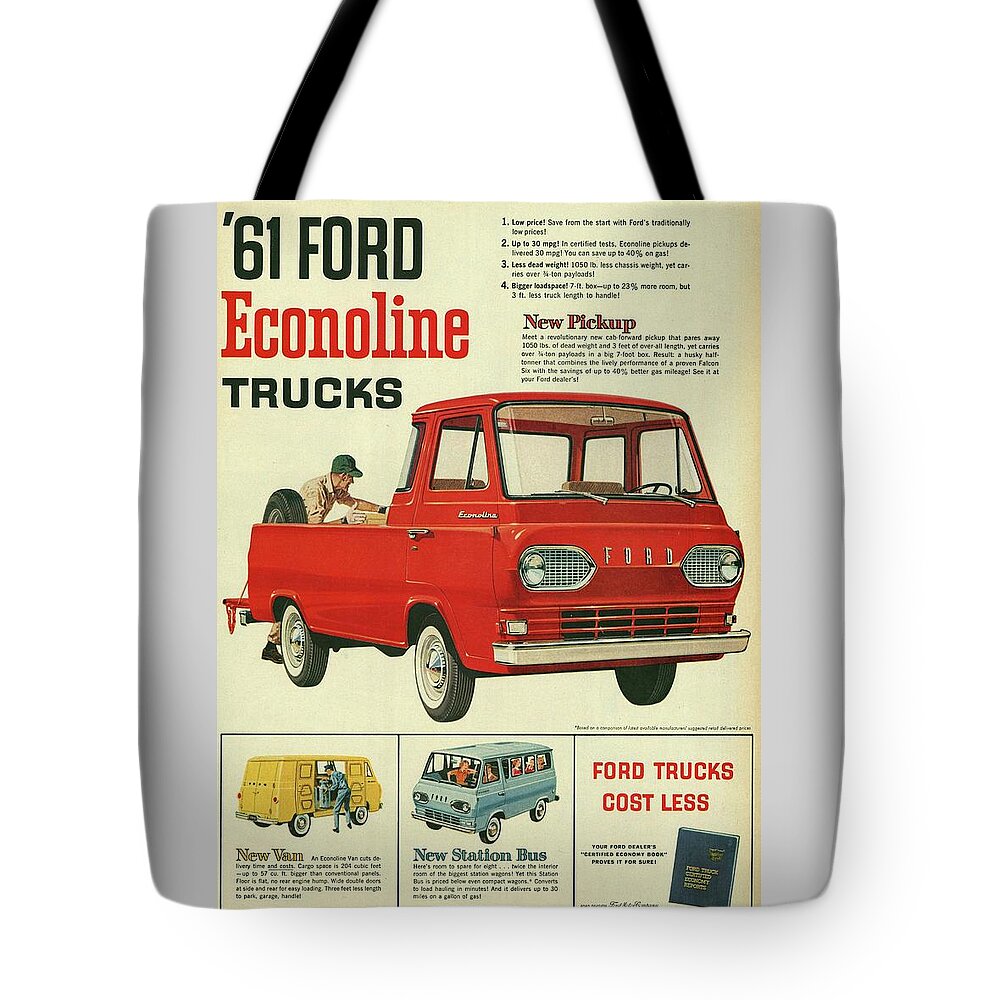The image depicts a white tote bag, against a solid white background, likely a digital mock-up suitable for a retailer's website. The bag features simple black handles, part of which is cropped off in the photograph. The front of the bag displays a vintage automobile advertisement, adding a retro flair. The advertisement is set against an off-yellow background and prominently features three Ford vehicles: a red pickup truck, a yellow van, and a light blue station bus. 

In the upper left corner of the advertisement, the text "61 Ford Econoline Trucks" is clearly visible. The red pickup truck, centrally positioned, is a two-seater with small black wheels and white wheel wells. The word "Ford" is emblazoned across its front, complete with a silver grill and headlights. A man wearing a hat and work shirt is seen in the truck bed, possibly loading or unloading cargo. Additional text about the truck's features appears in the top right corner, though it is too small to read clearly. Below the main image, there are three smaller squares, each providing further information about the truck. In the lower right corner, the text "Ford Trucks Cost Less" is prominently displayed beside a picture of a book.